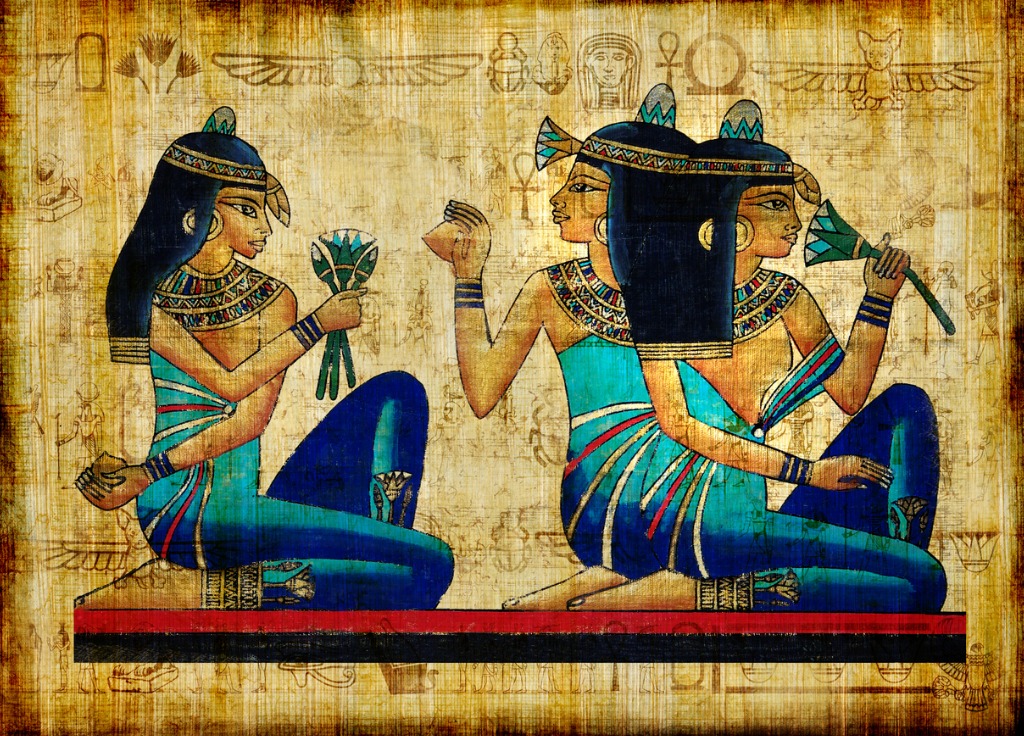The image depicts an ancient Egyptian painting, meticulously crafted on a sandy-colored parchment that has aged into tones of yellow and brown, reminiscent of a time-worn map. Dominating the artwork are three nearly identical women, richly adorned in vibrant blue and teal attire with intricate multicolored patterns, most notably around the neck and lower edges of their dresses. Each woman wears a matching intricately designed headband with a feather detail, and their dark hair is styled uniformly, accentuated by large golden earrings. The central woman on the left holds a decorative hand fan, while the women on the right, who appear extraordinarily close, almost conjoined, are each holding flowers in various stages of bloom. They sit gracefully on a low platform or rug, distinguished by its red top and black bottom. The background is filled with Egyptian hieroglyphs and symbols, including Ankh signs and stylized bird wings, adding depth and historical context to the scene. The overall composition blends muted and vibrant hues, emphasizing the women's ornate outfits against the aged, symbolic backdrop.